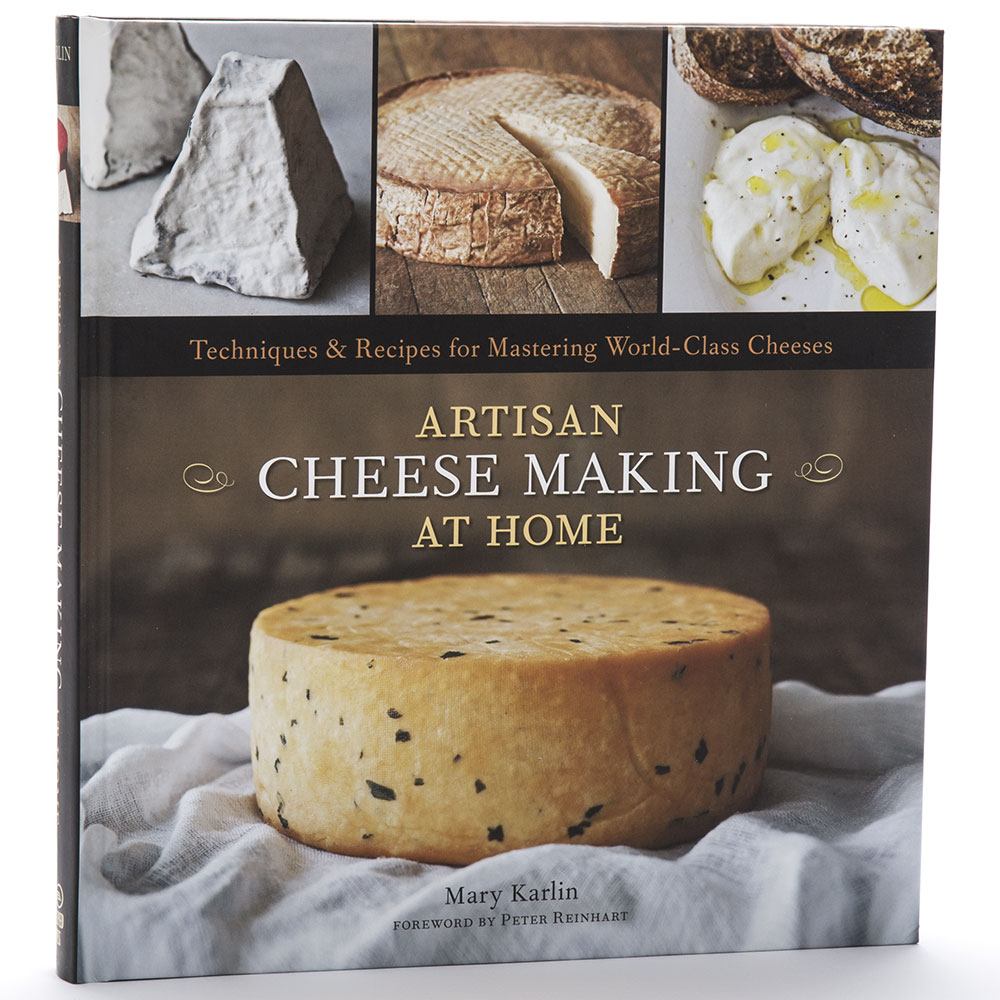This image showcases the front cover of the book "Artisan Cheese Making at Home" by Mary Carlin, with a foreword by Peter Reinhart. The cover is vertically oriented, providing a clear view of the detailed design elements. The title text is prominently displayed, with "Artisan" and "at Home" in gold lettering, while "Cheese Making" is in white. Below the title, a large, uncut cheese wheel occupies the center, characterized by its light brownish-yellow color with dark speckles embedded in it. This cheese wheel is laid atop a ruffled, off-white piece of fabric, adding a rustic touch to the presentation.

At the top right third of the cover, there are three smaller, distinct images of various cheeses arranged from left to right: the first shows a couple of white cheese wedges; the second displays a light brown cheese with a slice missing; and the third features a creamy, wet cheese drizzled with oil, possibly brie, served with toast pieces and sprinkled with black pepper. A banner between these images and the larger cheese wheel photo reads, "Techniques and Recipes for Mastering World-Class Cheeses," summarizing the book's content. The cover is slightly tilted against a white background, providing a clean, visually appealing presentation.